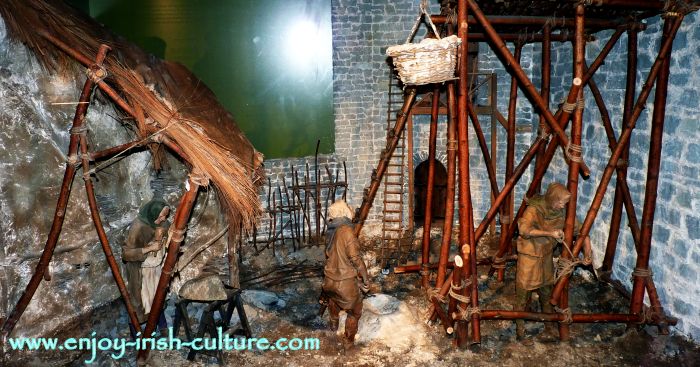The image is a detailed depiction of historical life in Ireland, presented as an exhibit at www.enjoyirishculture.com. The scene is set against a rough stone wall and features a wooden framework with a thatched lean-to on the left. Under the lean-to, a woman, possibly accompanied by children, finds shelter. In the middle of the scene, a hooded figure looks up at a wicker basket suspended from the wooden structure. To the right, another person is actively tying wooden pieces together, as if constructing the framework, perhaps for an outbuilding made from bamboo and rushes. The figures, dressed in plain, historical clothing with scarves over their heads, create a vivid portrayal of traditional Irish life, possibly from the 1700s or 1800s. The scene, which includes a stone fireplace and a ladder, is set on a dirt floor and intricately details the construction process of that era.